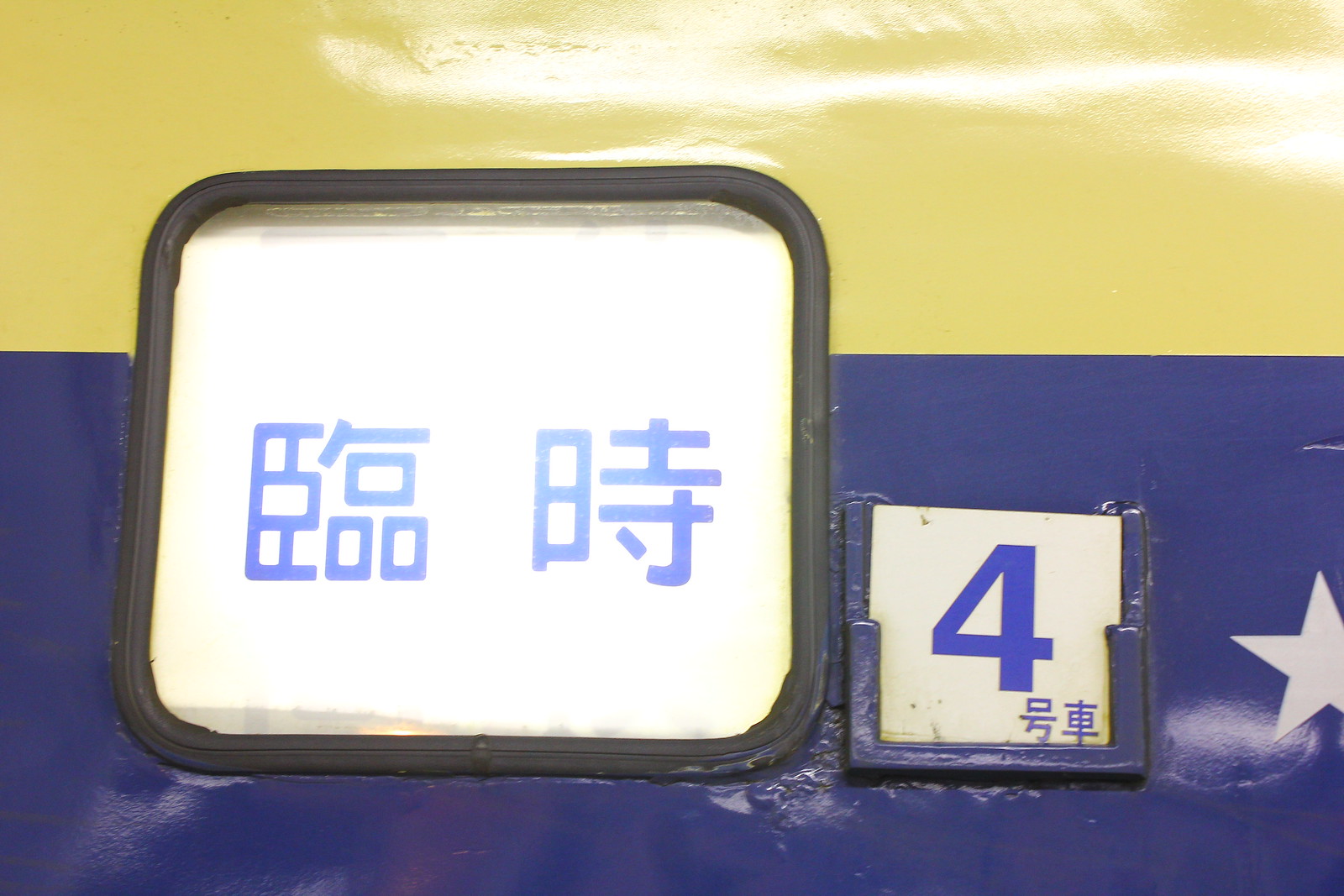The image showcases a close-up of a board with distinct colored strips: a golden yellow strip at the top and a purplish-blue strip at the bottom. In the lower right corner of the image, a white star is visible. The board features two white signs with peeling paint at the bottom. The sign on the left is a larger square with a black border, containing two blue Chinese symbols on a white background. To its right, a smaller square sign is partially bordered in blue and displays the number 4 in purple, with two Chinese symbols beneath it. The overall scene portrays a detailed and worn piece of signage against a visually striking blue and yellow backdrop.